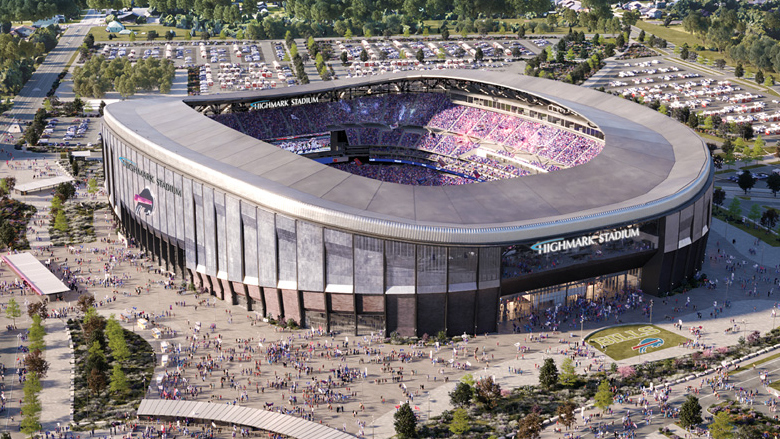The image showcases a detailed aerial view of Highmark Stadium, home to the Buffalo Bills, on a sunny day. The stadium, named Highmark Stadium in white lettering at the front, is a large oval structure with an open roof, allowing a clear view inside. The jumbotron inside the stadium displays ongoing sports action, with the stands packed to capacity, giving an impression of excitement and vibrancy. Outside, numerous tiny figures, resembling ants from the height, are seen moving around the concrete areas and entering the stadium. The front of the stadium features the "Bills" logo and emblem of a buffalo, etched prominently in a grassy area. Surrounding the stadium is a packed parking lot filled with cars, blending into a backdrop of scattered trees. Towards the front, there are additional details like tents in the grassy areas, possibly indicating tailgating activities. The entire scene is vivid, capturing the bustling atmosphere of a game day packed with passionate fans.